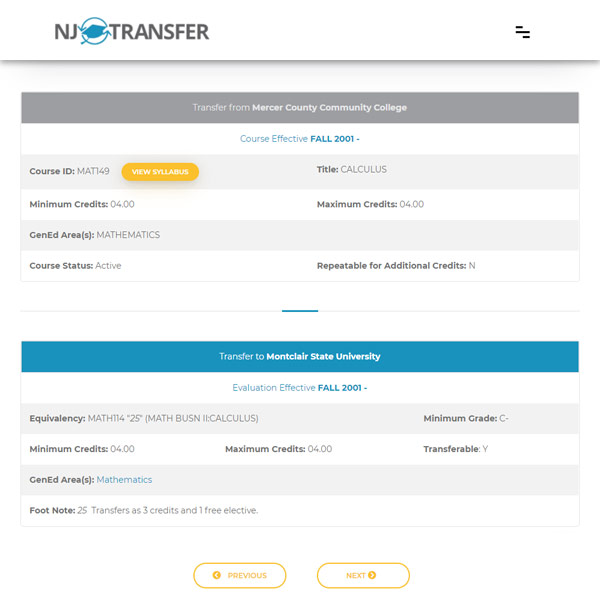Website Screenshot: NJ Transfer Detailed Information 

The image features a website page with the header "NJ Transfer". Situated between the words "NJ" and "Transfer" is a blue circle containing an indeterminate blue shape.

Beneath the header, a gray bar with white text reads, "Transfer from Mercer County Community College". Directly below this, in blue text on a white background, it states, "Course Effective Fall 2001".

Following this, another gray bar presents the bolded label "Course ID" in black font, followed by "MAT 149". Adjacent to this information is an orange push button labeled "View Syllabus" in white text.

Further down, the word "Title" in bold is displayed, with "Calculus" immediately below it. This is followed by a white bar where the black, bold text "Minimum Credits" states "04.00". On the right, the term "Maximum Credits" in black font also reads "04.00".

A gray bar beneath it emphasizes "Gen Ed Areas" in bold, followed by the word "Mathematics" in black font. Below this is a white bar displaying "Course Status" in bold black font, indicating the course status as "Active". Additionally, "Repeatable for additional credits" in bold, confirms with "N".

Moving further down, a blue bar with white text reads, "Transfer to Montclair State University" with "Montclair State University" in bold text. Below this, a white bar in blue font specifies "Evaluation Effective" and "Fall 2001" in bold.

The following section on a gray bar shows "Equivalency" in black font, revealing the content "Math 114" and "25" in quotes. Included is the detail "Math BUSN Calculus" and "BUSN 2 Calculus".

Adjacent information in bold black font indicates "Minimum Grade" as "C-". Underneath, a white bar shows the "Minimum Credits" as "04.00" and the "Maximum Credits" as "04.00" in bold.

Furthermore, "Transferable" is indicated with a bold "Y". The "Gen Ed Areas" section below in bold shows the emphasis on "Mathematics" in blue against a gray background.

At the bottom, a white bar labeled "Footnote" in bold contains the information: "25 transfers as 3 credits and 1 free elective".

The footer of the page features two navigational buttons: an orange outlined button labeled "Previous" with a left arrow, and another labeled "Next" with a right arrow, both in orange text.

This comprehensive description encapsulates all the visual and textual elements of the given website screenshot.